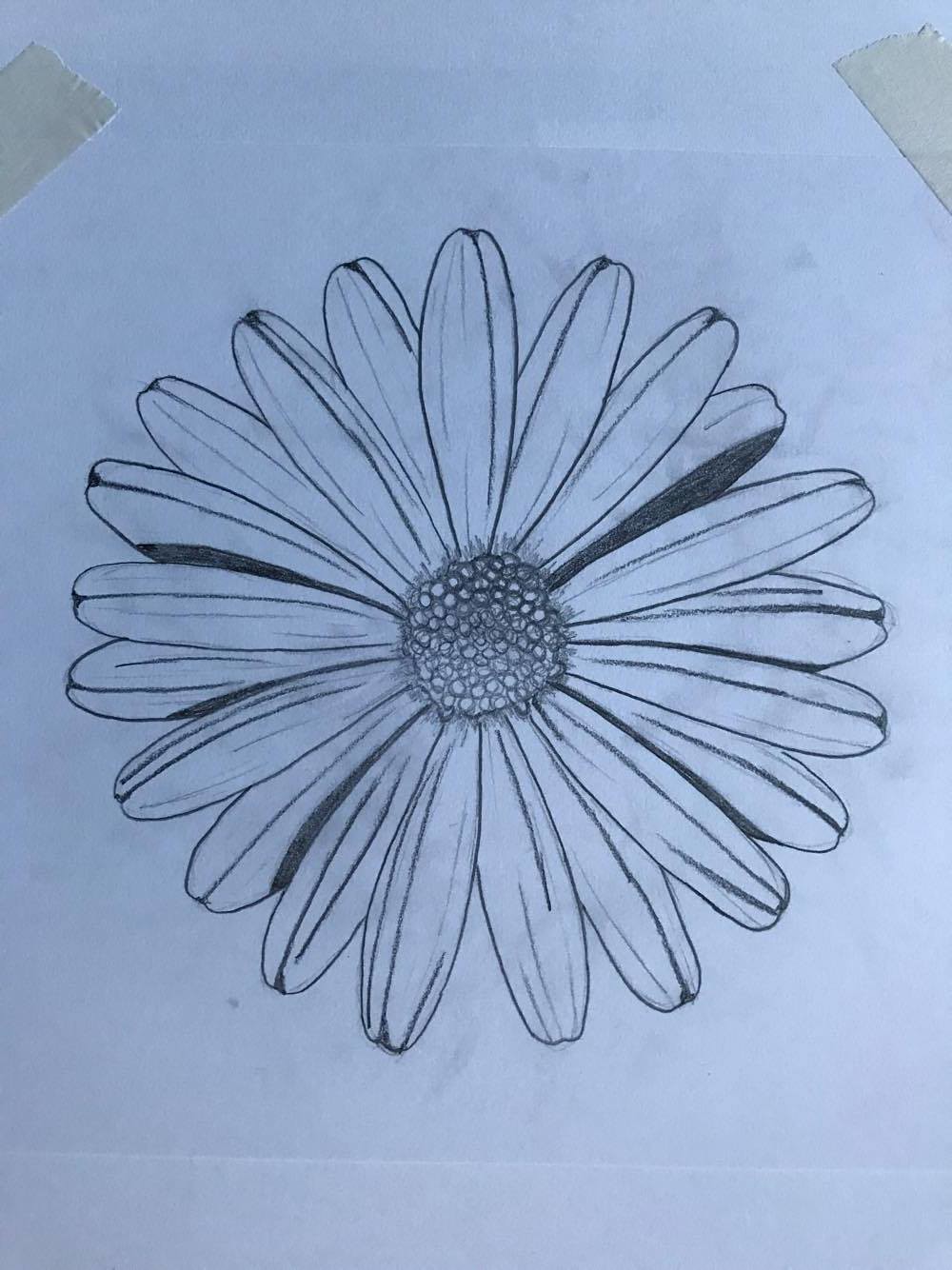This photograph captures a detailed black-and-white pencil or charcoal drawing of a flower with abundant petals. The image is focused directly on the bloom, showcasing its intricate design. The flower's center is densely packed with numerous tiny circular elements. There are no stems or leaves visible, emphasizing the flower's symmetrical beauty. The drawing is affixed to a larger piece of paper using two small pieces of masking tape at the top and bottom. The artist’s identity remains anonymous, as the artwork provides no signature or initials. The simplicity and elegance of the monochrome line drawing highlight the delicate details and craftsmanship of the flower.